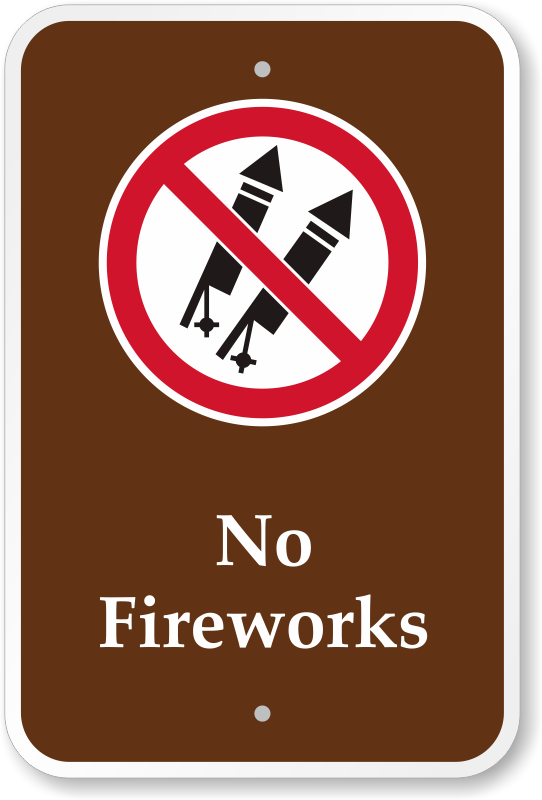This is an image of an informational sign, like one you might find in a park, designed to prohibit fireworks. The sign is vertically rectangular with rounded corners and has a thin white border surrounding a dark brown background. At the top and bottom center of the sign, there are small gray holes intended for mounting it onto a pole, fence, or wall.

Prominently displayed in the upper portion of the sign is a symbol indicating prohibition: a thin white circle surrounding a thicker red circle, which contains a diagonal red line crossing out two black silhouette images of rocket-style fireworks. These fireworks have a triangular top and a cylindrical base with a wick at the bottom.

Below the prohibition graphic, large white letters clearly state "NO FIREWORKS." The sign appears new and unused, ready for installation to prevent firework usage.